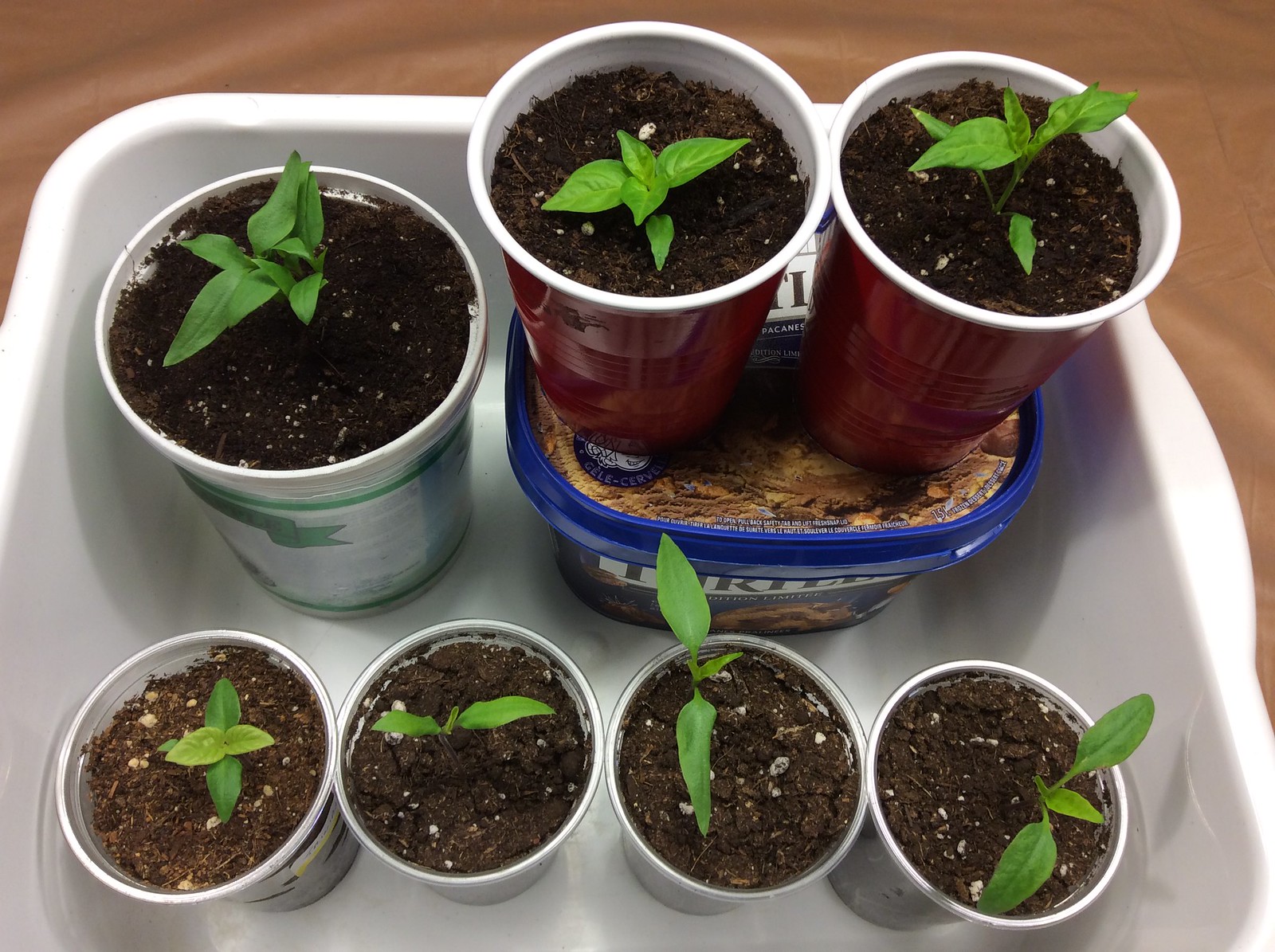In the image, a white plastic tub, resembling a dish tub, sits on a tan tablecloth. Inside this tub are seven containers, each holding sprouting plants with varying numbers of leaves. The front row consists of four white cups filled with soil to the rim, each nurturing small green sprouts at different stages of growth. Behind them, to the left, is a larger potted plant in an unidentified container, also filled with soil. To the right of this larger plant, there is a blue ice cream container supporting two red Solo cups. These cups too are filled with soil and have green sprouts emerging from them. The mixture of containers, including white cups, Solo cups, and possibly a yogurt container, adds diversity to the collection of young plants, which appear to be at various growth stages, possibly tomatoes or peppers.